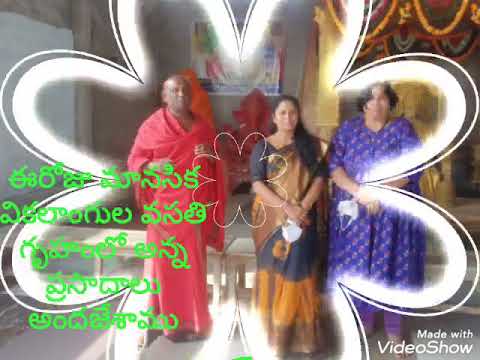In the square image, a photograph shows three people standing in the middle of a decorated room, surrounded by a creative white flower-shaped border pattern. The man on the left is bald and wears a long red robe. To his right are two women; the woman in the center is dressed in a black and yellow saree with long black hair, and the woman on the right wears a blue dress with a printed pattern and has short black hair. The background features an image of a Ganesh idol and flowers that adorn the room. The edited image includes five lines of text in a foreign language in green on the bottom left, and a watermark on the bottom right saying "made with video show" in white letters. The details on the faces are a bit blurry, making them hard to distinguish.